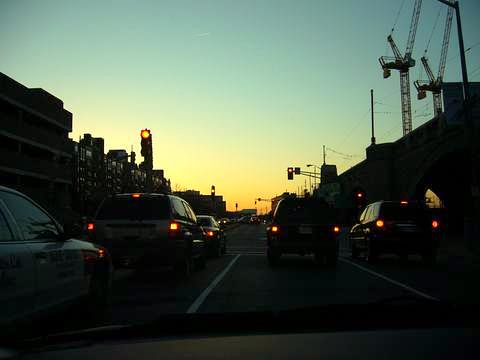This square color photograph captures a city street scene at dusk, taken from inside a car. The three-lane street is lined with cars: on the right lane, a single car is visible; in the middle lane, another car is directly ahead; and in the left lane, three cars are staggered, one slightly in front and two further ahead. The street is halted at a red light, while another red light farther down the road adds to the urban glow. The sky, transitioning from an orange sunset to a teal green horizon, casts a dim light that makes the red brake lights of the cars particularly vivid. On the right side of the image, beyond some darkened buildings, large construction cranes tower into the sky, suggesting ongoing development. The left side of the street features indistinct brown and black buildings with scattered windows, potentially apartment complexes. The overall scene is marked by an intriguing blend of urban activity and the serene colors of the fading day.